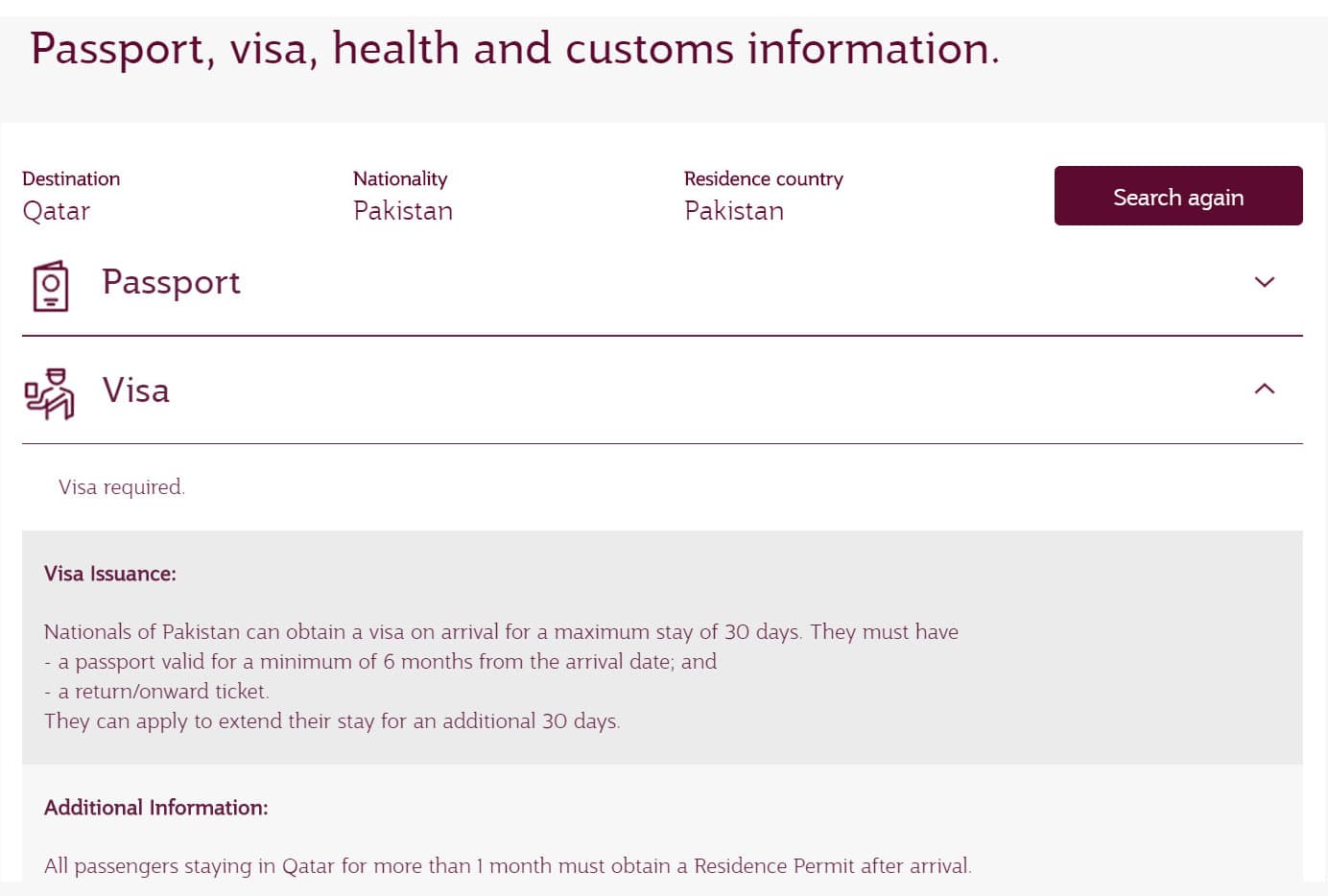This is a screenshot of a web page providing essential travel information. At the top, a gray banner contains the text "Passport, Visa, Health, and Customs Information" in bold black font. Directly beneath this banner, a white section displays crucial details in black font: 

- **Destination:** Qatar
- **Nationality:** Pakistan
- **Residence Country:** Pakistan

Under this white section, there is a black rectangle with white text that reads "Search Again."

Further down, the page lists specific sections related to travel requirements:

1. **Passport:** Accompanied by a small icon of a passport.
2. **Visa:** Represented by an icon of a person holding a cup. Following this, the text reads "Visa Required" in gray font.

Below this is a gray rectangle containing detailed visa issuance information in black font:

- Nationals of Pakistan can obtain a visa on arrival for a maximum stay of 30 days.
- To qualify, they must possess a passport valid for at least six months from the date of arrival and a return or onward ticket.
- There is an option to apply for an extension to extend their stay for an additional 30 days.

At the bottom of the page, an "Additional Information" section notes:

- Passengers planning to stay in Qatar for more than one month must obtain a resident permit after arrival.